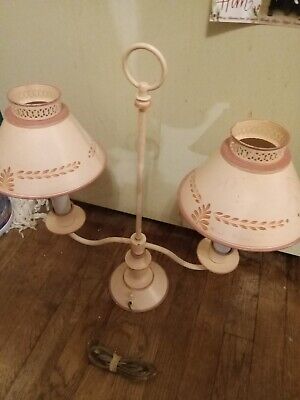This color photograph, taken in portrait orientation, focuses on a vintage lamp set against a beige wall. The lamp stands tall and narrow with a central post culminating in a rounded hook at the top. It features two curved arms, extending to the left and right, each ending in candelabra-style bases partially visible under conical light pink shades. These shades are adorned with a fern pattern in a darker pink beige color near the bottom, and have a fluted or painted motif around their tapered tops. An electrical cord is coiled at the lamp's base. The lamp is situated on a brown hardwood floor, and there are no other objects or decorations in the background, highlighting the lamp as the focal point of the image.